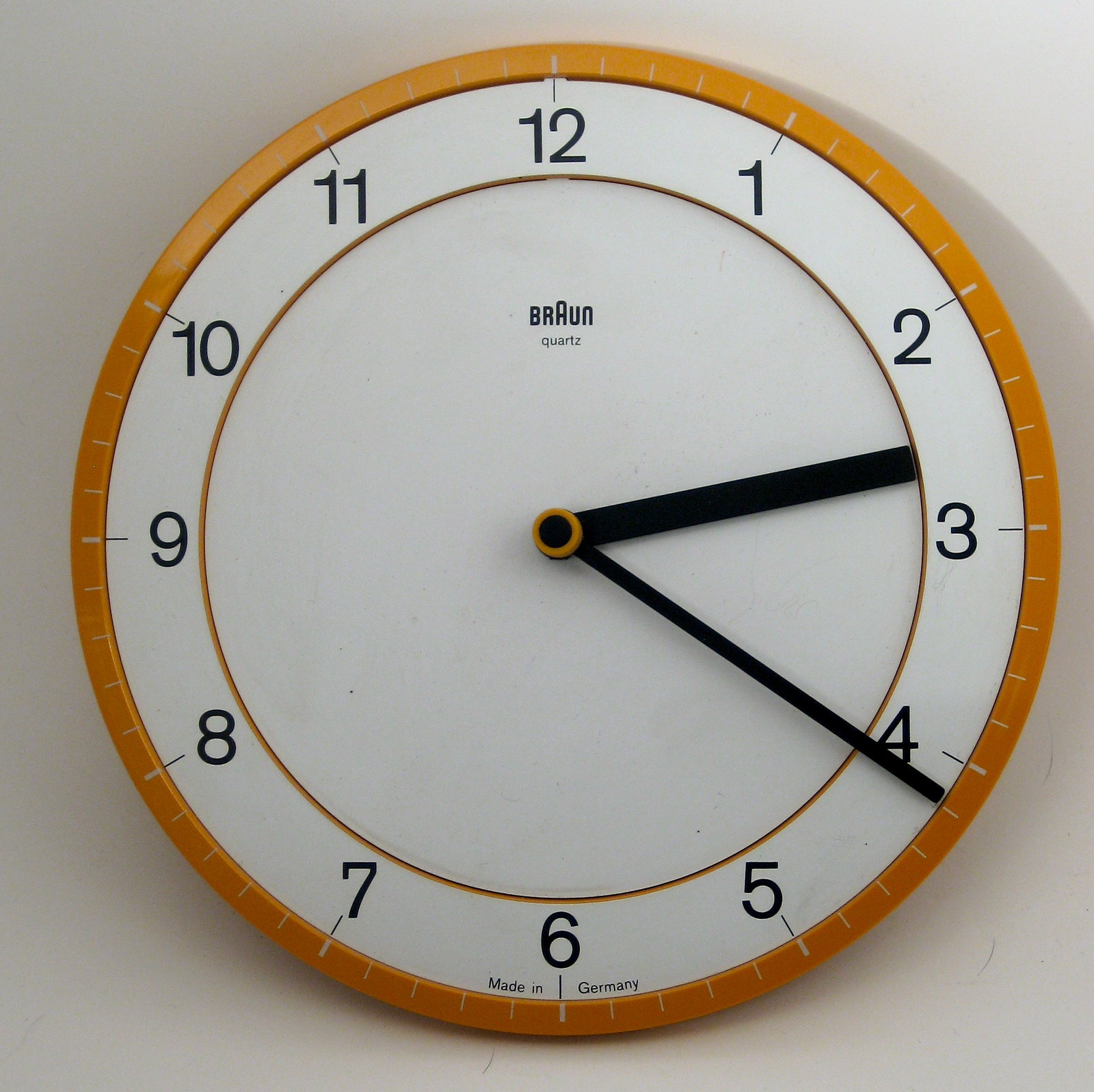This indoor photograph showcases a close-up of a wall-mounted round clock. The clock is centered against a plain white wall, drawing immediate focus to its simple yet striking design. The outer rim of the clock features a deep orange hue, which contrasts sharply with the pristine white clock face. Bold black numerals clearly mark each hour, making the time easily legible. The hands of the clock, also black, indicate the time as a few minutes past 2:20, specifically around 2:22. At the top of the clock face, just below the 12 o'clock position, the brand name "Braun" is inscribed, accompanied by the word "quartz." At the very bottom of the clock face, beneath the number six, the phrase "Made in Germany" is written, subtly emphasizing the clock's origin and craftsmanship.